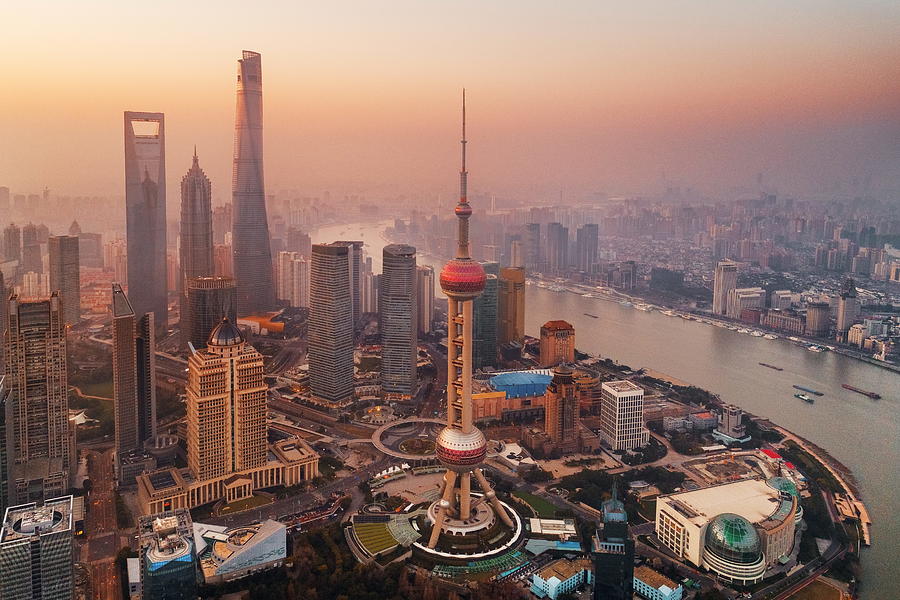This aerial photograph, likely taken over an American city, prominently features a distinctive spire with a pointed top. The spire is adorned with three conspicuous red structures cascading downward, with the third segment—near the base—exhibiting a mix of white and red colors. The base itself is unique, comprising circular sections supported by a tri-point standing structure. The cityscape is densely packed with a variety of buildings, resembling a Tetris game, predominantly on the left side of the image. These structures range from medium to tall skyscrapers. On the right side, a winding river bisects the city, curving elegantly as it flows downwards in the picture. Numerous boats and potential cargo ships can be seen navigating the river, which appears to separate the sprawling urban landscape into two distinct areas populated with buildings, roads, and more city features.